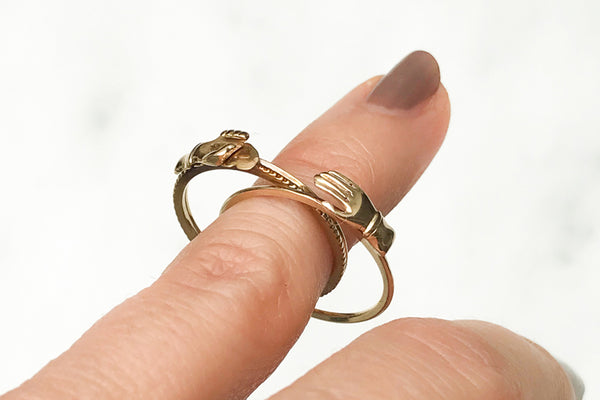The photograph showcases a female's finger, prominently displayed against a white background, emerging from the bottom left corner and pointing towards the top right. The focal point is the woman's pointer finger, adorned with two intricately designed gold-plated rings. The lower ring features a hand design, while the upper ring, appearing slightly angled and harder to discern, seems to depict another hand or possibly a foot. This creates a layered, concentric effect on the finger. The rings are cleverly designed to hook onto the finger without the need for sliding. The finger's nail is long, painted with a brownish color, and shows signs of chipping near the cuticle. Adjacent to the adorned finger, another finger is also faintly visible, pointing towards the lower right-hand corner.